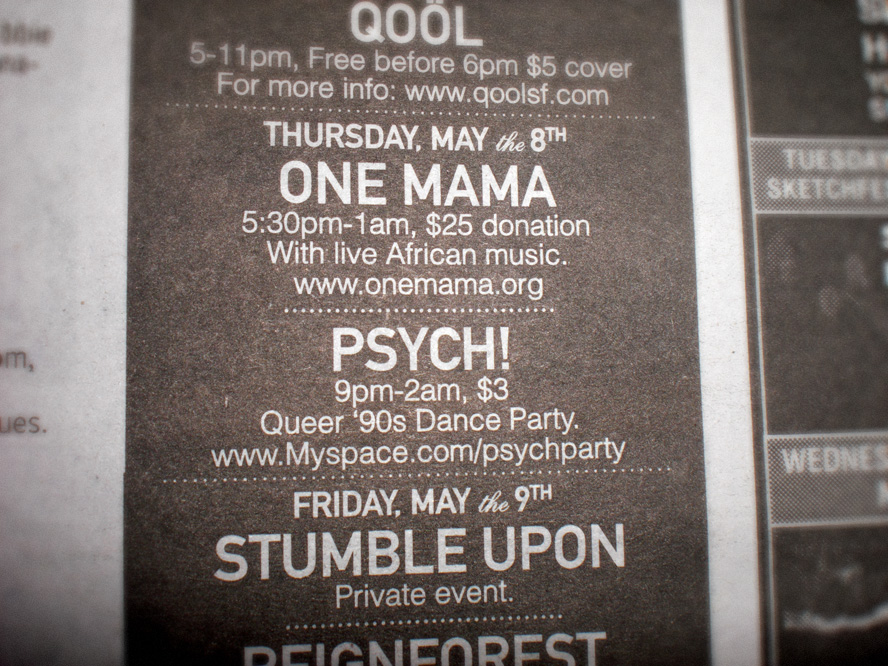The image depicts a black-and-white section of a newspaper or magazine, characterized by a slate gray background with white text. The layout includes a dark column divided into sections by horizontal dotted lines, detailing events at a musical venue named QOOL. At the top, an event is listed for Thursday, May 8th, featuring "One Mama" with live African music, running from 5:30 p.m. to 1 a.m., suggesting a $25 donation. More information can be found at www.qoolsf.com and www.onemama.org. Another event is listed the same day from 9 p.m. to 2 a.m. called "Psych!" This is advertised as a Queer 90s Dance Party with a $3 cover charge. On Friday, May 9th, the venue hosts "Stumble Upon," marked as a private event themed around a rainforest.